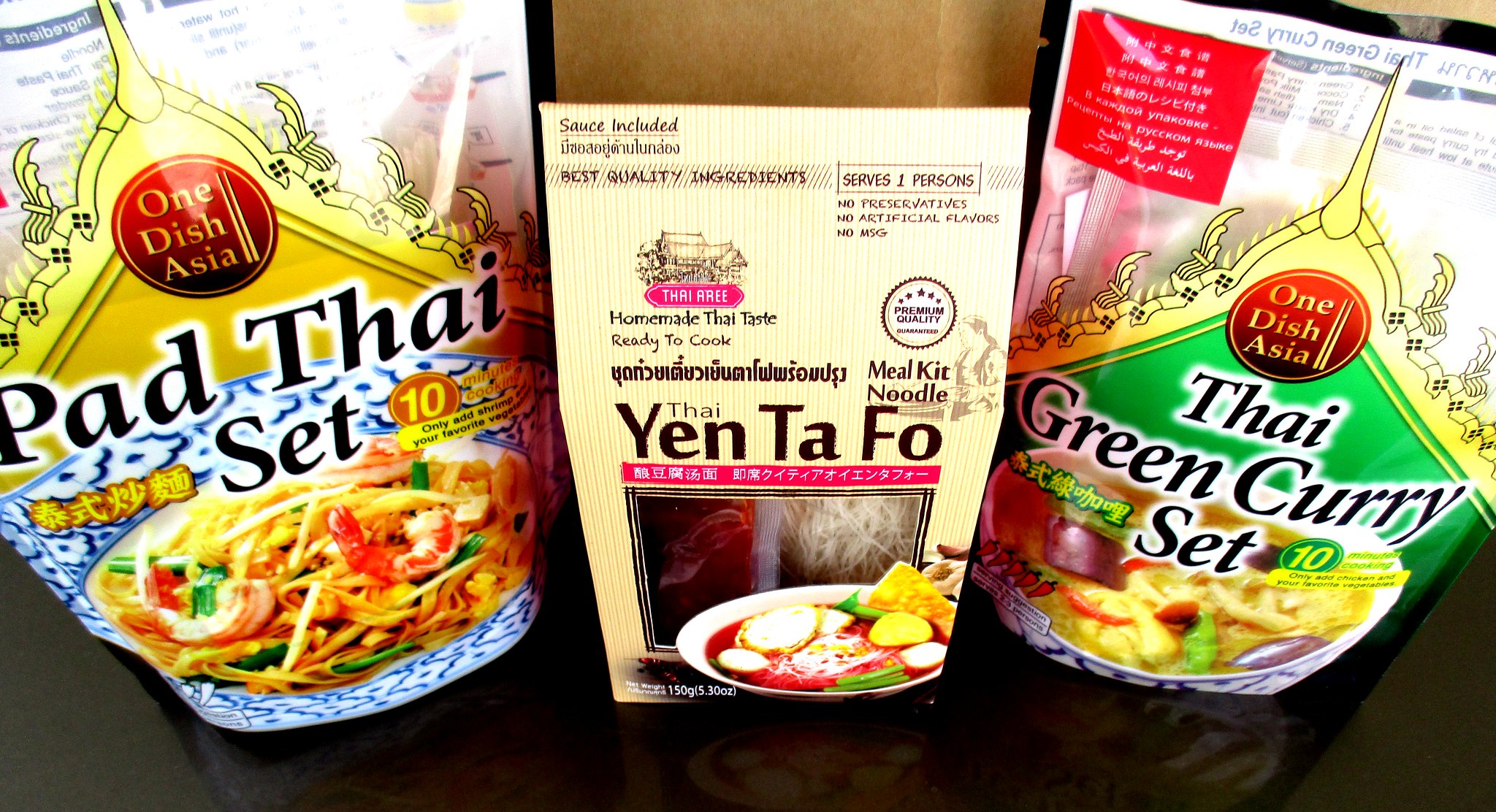The horizontal rectangular image features three packages of oriental food products on a black surface. On the left, there's a colorful bag labeled "Pad Thai Set" with the brand logo "One Dish Asia." The packaging, in gold, blue, and white, depicts shrimp Pad Thai and carries a red circle highlighting "One Dish Asia." The package appears to be made of heavy plastic. In the center, there is a simpler paper box labeled "Thai Yen Ta Fo Meal Kit Noodle." It has a viewport displaying uncooked seasoning and noodles, and features an image of the dish on the front. On the right, another "One Dish Asia" package showcases a "Thai Green Curry Set" with predominantly gold, green, and white colors. The packaging illustrates a bowl of Thai Green Curry, featuring what appears to be noodles along with purple and green food items. All packaging includes Thai writing and emphasizes authentic homemade Thai taste.